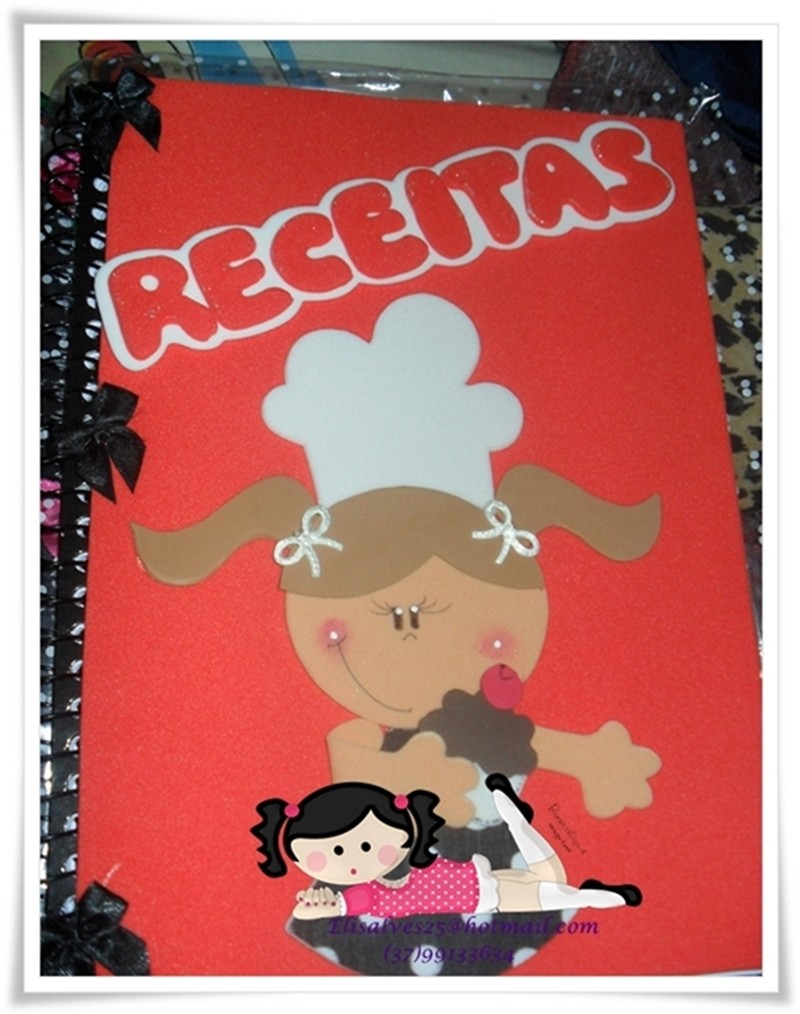The image showcases a vibrant, stylized cover of what seems to be a recipe book titled "Receitas," spelled out prominently in red letters on a white background at the top. The book cover is predominantly red with black spiral binding running along the left side, accented by three evenly spaced yellow ribbons. Central to the cover, a large illustration features a girl with a cheerful expression, rosy cheeks, and brown hair tied into pigtails with white bows. She wears a white chef's hat, emphasizing the culinary theme. Directly below her, there's a whimsical drawing of a cupcake adorned with a cherry on top. Positioned at the very bottom, another playful illustration depicts a smaller girl lying on her tummy, legs kicked up, dressed in a red and white polka dot dress with black shoes and white socks. Additionally, the email "LisaAlves25@hotmail.com" can be found on the cover, suggesting a personal touch. All elements are arranged meticulously to create an inviting and fun aesthetic for the recipe book.